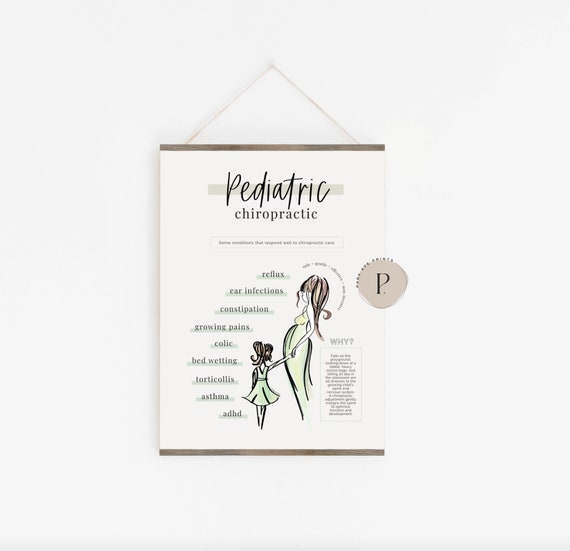The photo shows a sign hanging from a white wall, likely in a doctor's office, promoting pediatric chiropractic care. The sign, printed on sturdy stock and measuring about 8.5 by 11 inches, features the words "pediatric chiropractic" in an elegant script and serif font at the top. Below this, an illustration of a pregnant woman holding a little girl's hand is prominently displayed. The sign lists various conditions that can be addressed through chiropractic care, including reflux, ear infections, constipation, growing pains, colic, bedwetting, torticollis, asthma, and ADHD. On the right-hand side, there's a light beige or gray circle with the letter 'P' inside it, resembling a seal. Beneath the list of conditions, a box labeled "Why?" suggests there is additional information explaining the benefits of pediatric chiropractic care, though the smaller text is not legible. This sign emphasizes the potential health benefits of chiropractic therapy for children, aiming to educate parents and caregivers.